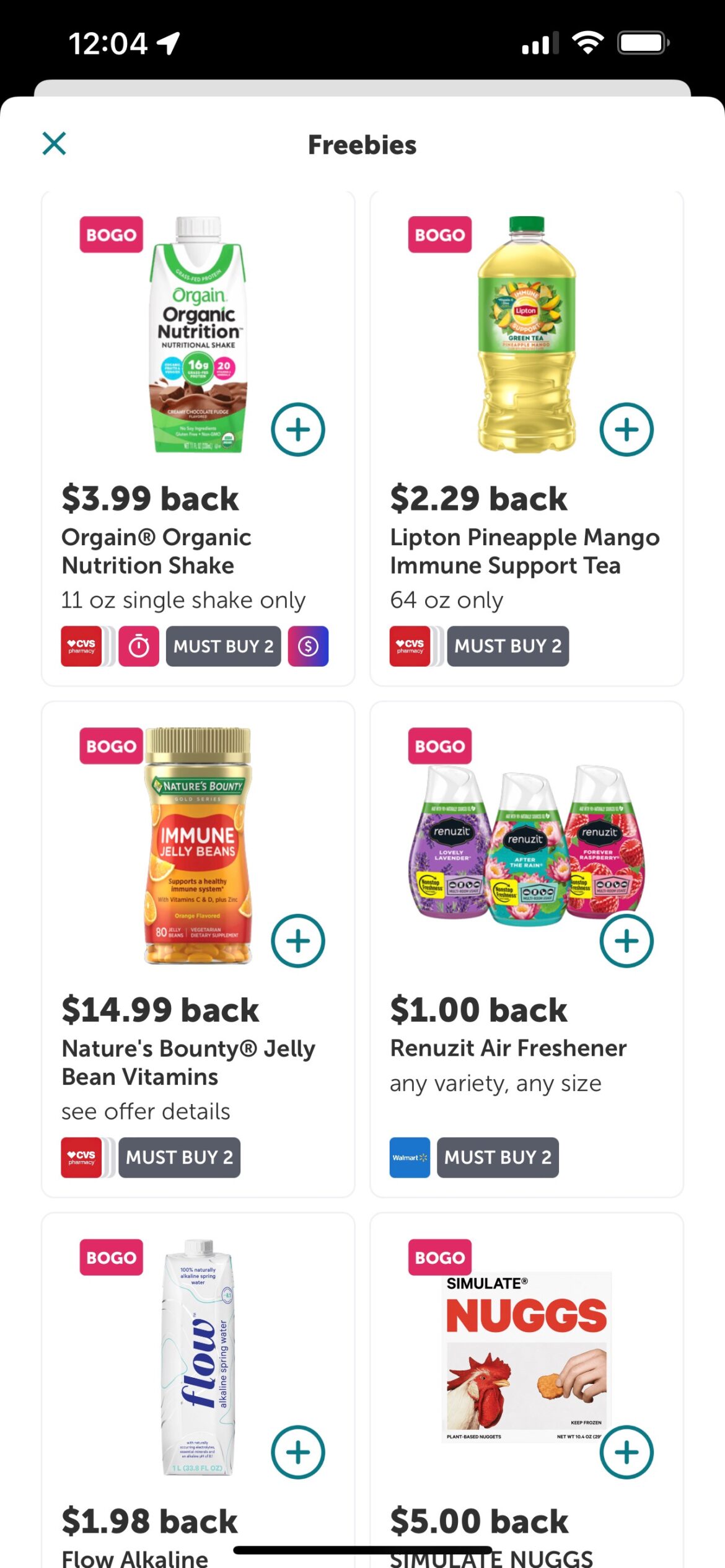Here is the revised and detailed caption:

---

This iPhone screenshot displays an app interface at 12:04, as indicated by the time in the upper left corner, with a solid battery icon on the right, showing a strong connection with three illuminated bars in blue.

The interface appears to be advertising various food, drinks, and other items. At the top, a space for freebies is available for users to click on, alongside an 'X' icon on the left to possibly close the section.

Featured items include:
1. Orgain Organic Nutrition Shake
2. Lipton Pineapple Mango Immune Support Tea
3. Immune Jelly Bean Vitamins
4. $1 back on any variety, any size of Renuzit Air Freshener
5. $1.98 back on Flow Alkaline Water
6. $5 back on Simulate Nugs

Each item has a blue circle with a plus sign, indicating that users can click to select the offer. The first four items note that the user must buy two to qualify for the offer. Below these items, there are miscellaneous images such as a red box with text inside, a red box with a circle, and an arrow, suggesting additional interactive elements. The last two items do not display any stipulations, although this could be due to the image being cut off.